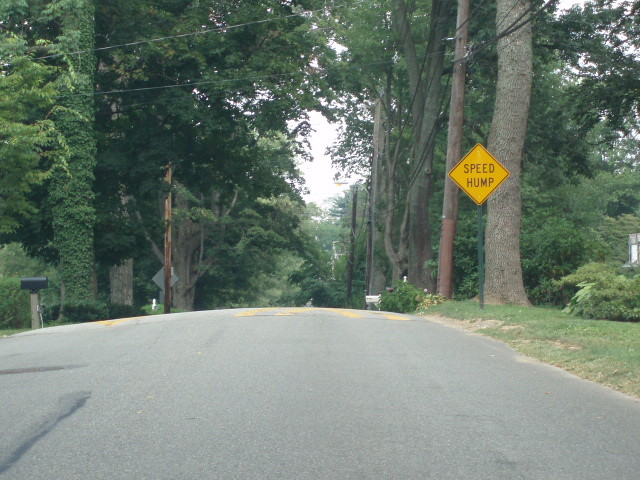A quiet residential street stretches out in front of the viewer, with the black asphalt contrasting sharply against the green surroundings. On the right-hand side, a yellow diamond-shaped "Speed Hump" sign is prominently displayed on a green pole planted in the grass, warning drivers of upcoming road conditions. The street is lined with tall, lush trees, their branches heavy with vibrant green leaves, creating a serene and verdant canopy. There is no traffic visible, adding to the peaceful nature of the scene. A white mailbox stands on the right edge of the frame, serving as a subtle landmark in this tranquil neighborhood setting. The photograph is taken from a slightly inclined angle, providing a clear but slightly angled view of the street that stretches ahead.